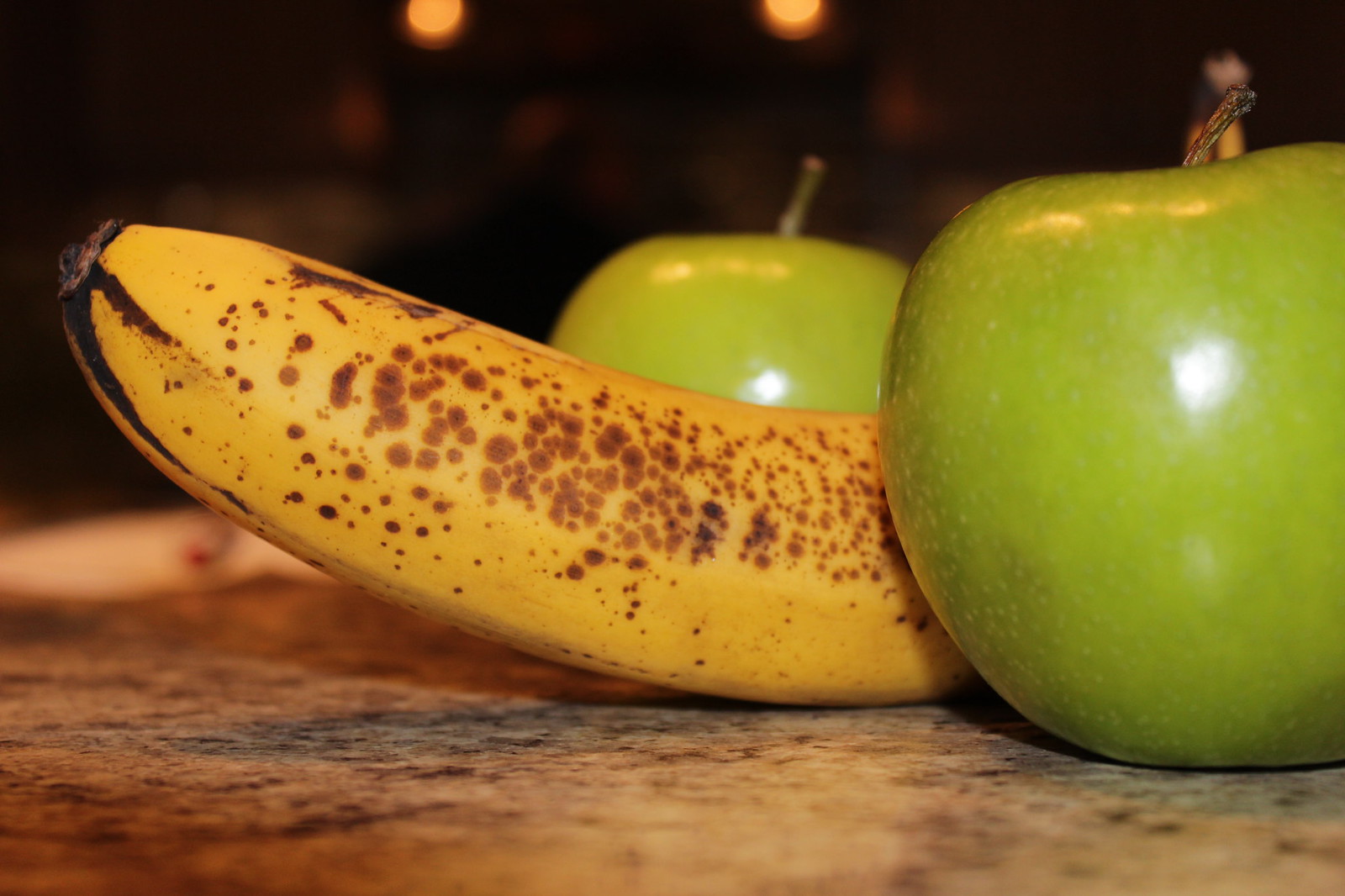On a mottled light and dark brown countertop, possibly made of faux marble or Formica, sits a ripe banana and two fresh green apples. The banana, positioned centrally, shows signs of ripening with a blackened tip and numerous brown spots, some of which are turning black. Flanking the banana on either side are two green apples, their waxy skins reflecting the bright light from the photographer's setup. The apples' stems are still attached, adding a touch of natural detail to the composition. The overall scene is well-lit, emphasizing the textures and colors of the fruit against the countertop's intricate pattern.